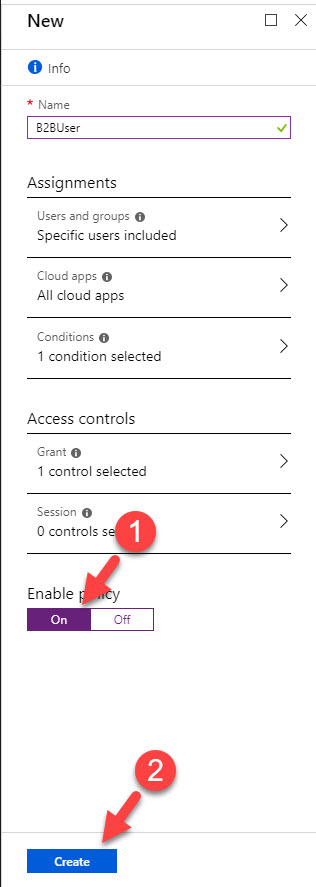This image portrays a detailed tutorial for utilizing a specific app, evidenced by a screenshot of the first page. In the top left corner, the word "New" is prominently displayed. Adjacent to this, an info icon is visible, followed by various input fields and settings.

The first input box is labeled "Name" and already populated with "B2B user." Below this are several categorized sections:
- **Assignments:** Specifies "Users and Groups," with "Specific Users Included" noted.
- **Cloud Apps:** Indicates "All Cloud Apps."
- **Conditions:** Mentions that one condition is selected.
- **Access Controls:** Highlights "Grant," with one control selected.
- **Session:** Lists zero controls.

Additionally, there are two toggle buttons labeled "Enable Privacy," offering an "On" or "Off" option. A prominent red button marked with the number "1" and an arrow directs users to select the "On" option.

At the bottom of the screenshot, a gray "Create" button is present. Above this button, there is another red button numbered "2" with an arrow pointing to the "Create" button, signaling that this should be the second step in the sequence.

This structured layout and visual aids ensure users can easily follow along and perform the steps as intended.